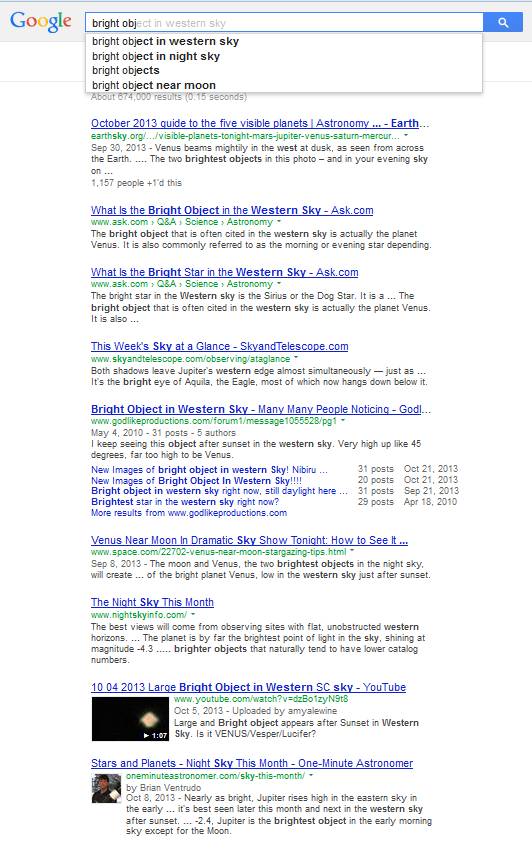A screen capture displaying a Google search results page for the query "bright object in western sky." At the top, the Google search bar prominently displays the input text, with "bright object" partially highlighted in black and the rest in a shadow gray. Below the search bar, a dropdown menu suggests related search queries such as "bright object in western sky," "bright object in night sky," "bright objects," and "bright objects near moon." 

Beneath the dropdown, approximately seven to ten search results are listed. The first result is titled "October 2013 guide to five visible planets," followed by "What's the bright object in the western sky" and "What is the bright star in the western sky," among others. Each search result includes a brief description and a clickable link.

The page design appears to be an older version of Google's interface, suggesting that the screen capture might be from a computer using a Google layout common around 2013 or earlier. This is further evidenced by the dates on the articles, which are all from 2013 or before.